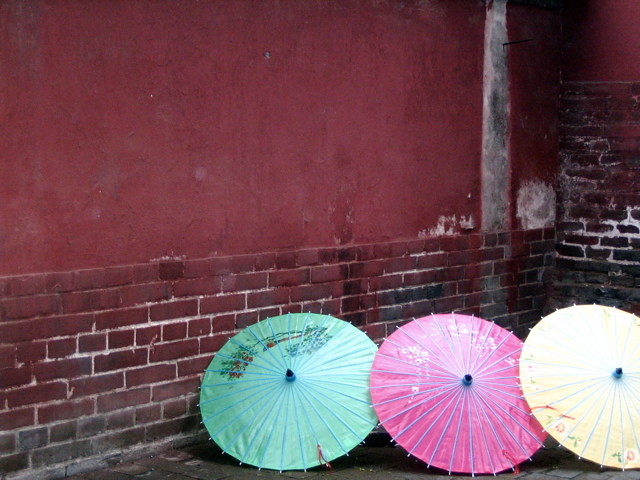This detailed photograph captures a vividly artistic scene set in an alleyway. The backdrop consists of a messy red wall and intersecting concrete and brick walls, which are painted a smudged burgundy red, with the bricks appearing worn and dirty. The concrete floor, reflecting the dilapidated ambiance of the setting, cradles three large, oriental-style umbrellas, reminiscent of the small decorative ones in exotic drinks but scaled up to functional sizes for rain protection. Facing the viewer with their tips touching, the umbrellas form the centerpiece of the image. They come in three colors: a mint seafoam green (Tiffany blue) with a floral pattern, a pink one adorned with white flowers, and a pale yellow umbrella also decorated with white flowers, each featuring a blue lining around the edges. This striking composition, void of any text, emphasizes the vibrant umbrellas against the gritty, textured backdrop, highlighting the contrast between the colorful elegance of the umbrellas and the shabby conditions of the alley.